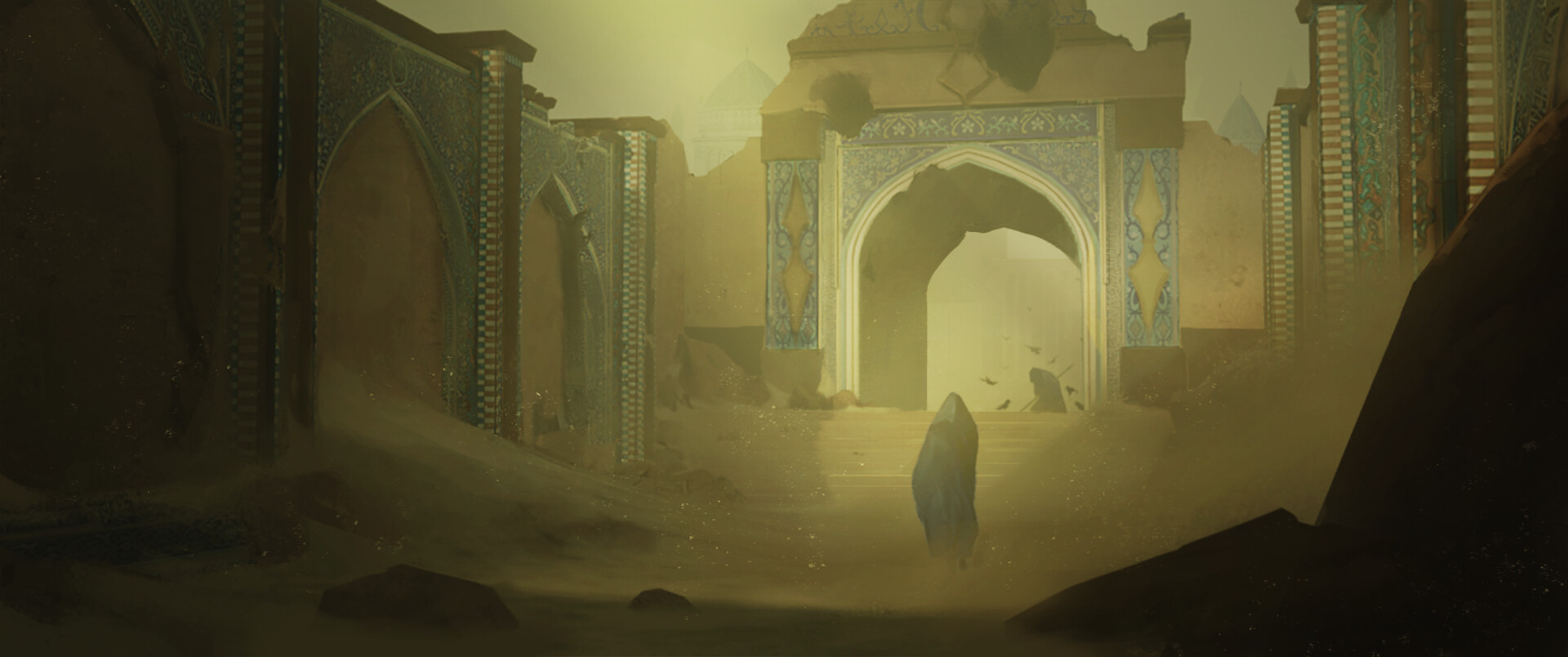In this screenshot of a video game, the scene depicts a vast, deserted temple laden with architectural grandeur, reflecting a blend of Biblical and ancient Islamic influences. The ominous atmosphere is accentuated by dust and debris filling the room, giving it a blurred, brownish, and foggy appearance as if engulfed by a sandstorm. The temple's majestic pillars and walls, adorned with intricate golden and blue pastel designs and patterns, speak of its former glory, though now in ruins. Dominating the scene is a lone, hooded figure draped in a black robe, reminiscent of the Grim Reaper, standing solemnly in a central position as if in prayer. Above this figure, an aura effect can be seen. To the left, a grand sword hangs on the wall beside a domed archway with steps leading up to it, hinting at an exit. Scattered rocks and stones further contribute to the desolate feeling of the scene. In the background, additional structures with large, ornate columns rise against a cloudy sky, reinforcing the sense of an ancient, forsaken place.